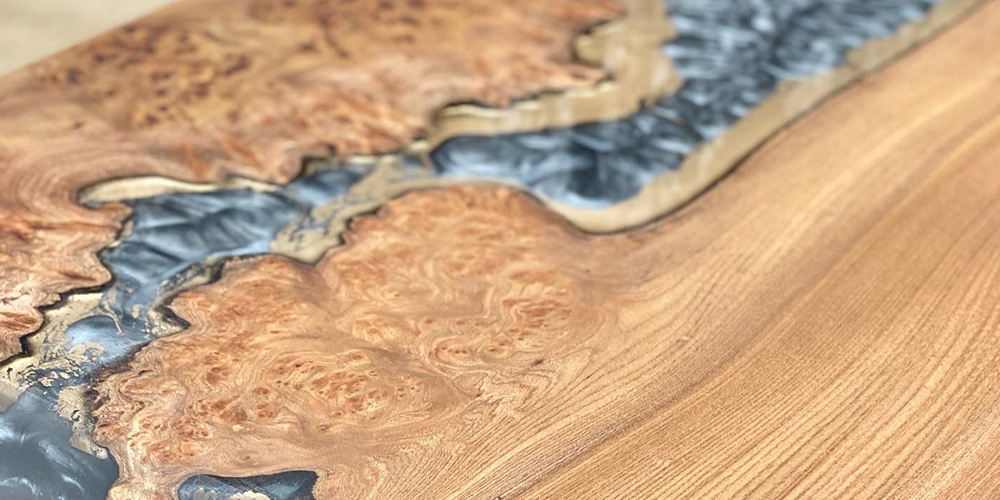The image showcases a detailed wood surface that appears reminiscent of a finely crafted tabletop. The wood, primarily light brown with patches of darker and lighter grains, has a series of intricate, natural lines and swirls that are typical of freshly sawn timber. Notably, there are segments of the wood adorned with inlaid materials that resemble resins or metals like silver or pewter, contributing a navy blue or bluish-gray hue. This inlay, flowing through the wood grain much like a river through a valley, gives the appearance of melted or poured metal, creating a textured, almost bubbled effect. The surface is further embellished with an off-white cream color in the top left corner and black and white lines, possibly imprinting or grooves, that add to the complexity of the design. These elements combine to give the wood an abstract painting-like quality. Although no text is present in the image, and there's no indication of a glass overlay, the composition is visually striking and highly detailed, suggestive of both natural artistry and crafted elegance.